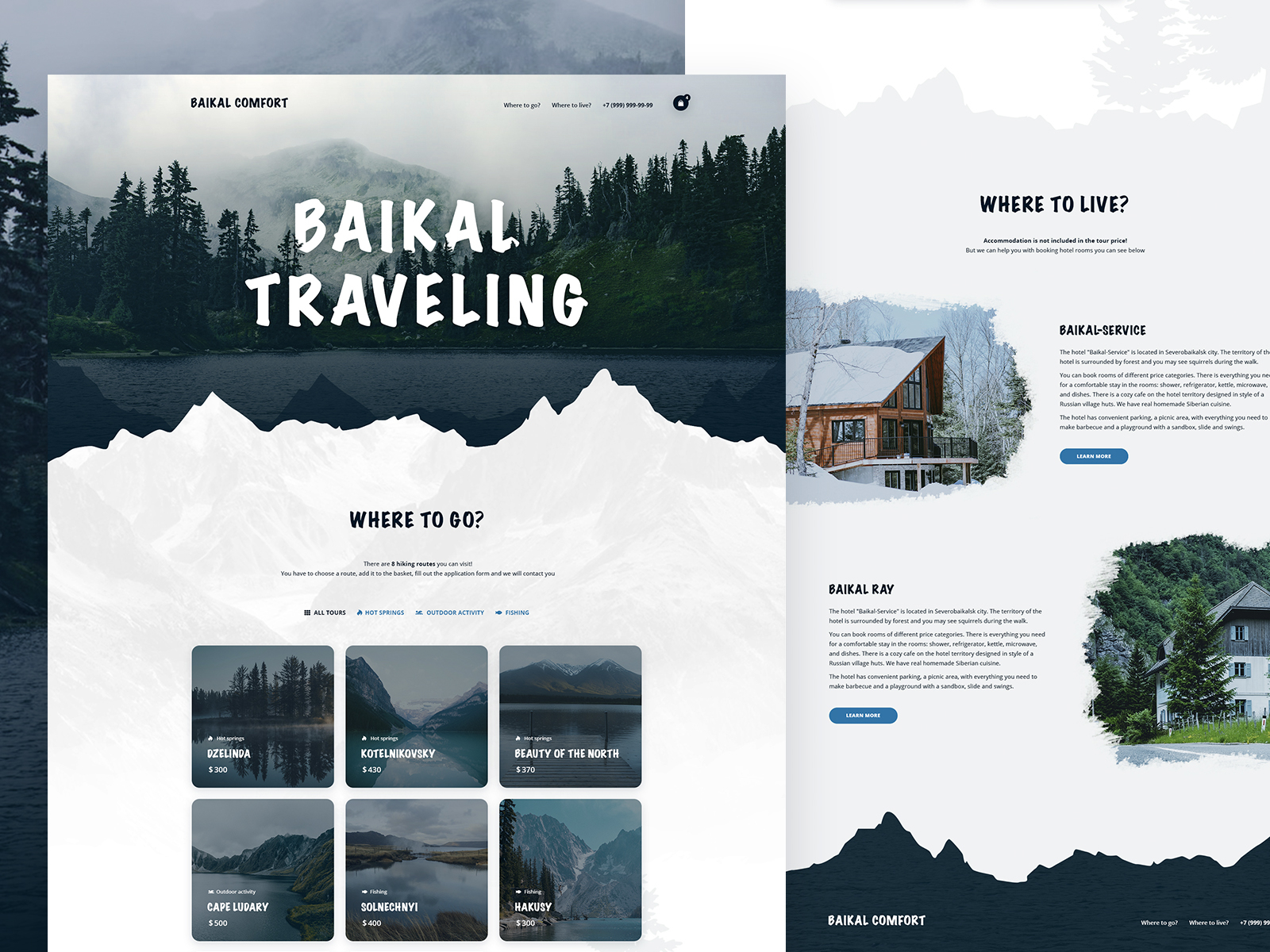This image comprises two distinct screenshots from a website detailing a travel service. At the topmost part of the image, the title "Baikal Comfort," spelled B-A-I-K-A-L Comfort, is prominently displayed. Underneath in bold white letters, it reads "Baikal Traveling." The central part of the screenshot features an evocative image showcasing a majestic mountain, a serene mid-ground populated with trees, and a picturesque lake adorned with snow in the foreground. The text "Where to Go" is prominently displayed below.

The section "Where to Go" showcases six enticing destination options presented in a grid format. The first row includes:
1. Dzelinda, spelled D-Z-E-L-I-N-D-A.
2. Kotelnikovsky, spelled K-O-T-E-L-N-I-K-O-V-S-K-Y.
3. Beauty of the North.

The second row includes:
4. Cape Ludar, spelled L-U-T-E-R-Y.
5. Solnechny, spelled S-O-L-N-E-C-H-N-Y-I.
6. Hakusy, spelled H-A-K-U-S-Y.

Each destination is illustrated with scenic views, typically featuring mountains and bodies of water.

On the right-hand side of the screenshot, a section titled "Where to Live" details accommodation options, noting that accommodation is not included in the tour price. The first option listed is "Baikal Service," spelled B-A-I-K-A-L hyphen Service. This choice is accompanied by an image depicting a cozy cabin nestled in the snow, complete with a spacious porch and balcony, set against a backdrop of mountains. The second accommodation option is "Baikal Ray," accompanied by an image of a forest and a mountain standing beside a white and gray three-story house or apartment building.

At the bottom of the screenshot, an image featuring mountain peaks is visible, with the text "Baikal Comfort" overlaid.